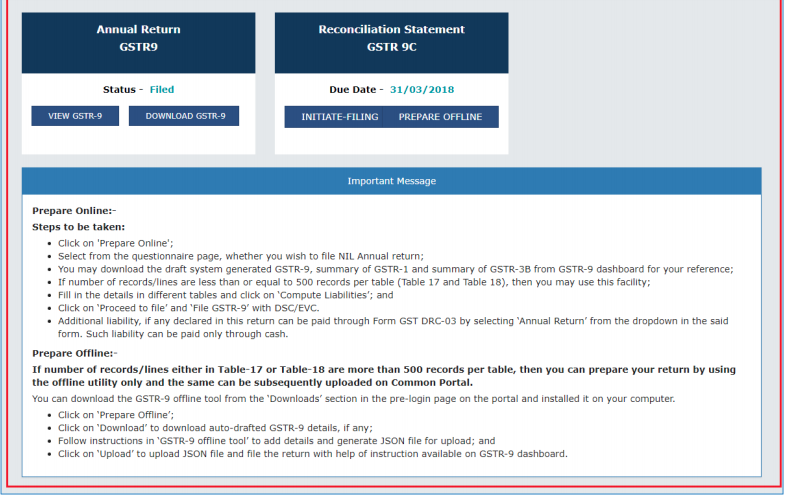The image showcases a website with a light gray background, bordered by a thin red line on the left, right, and bottom edges. At the top of the page, there are two prominent sections.

The first section features a white square labeled "Annual Return" in capital letters. Beneath this label, it reads "GSTR 9" followed by the status "Filed." Two options are available here: "View GSTR-9" and "Download GSTR-9."

Adjacent to it, the second section is a dark blue banner with white text. It displays the heading "Reconciliation Statement" in capital letters, followed by "GSTR 9C." The due date "31-03-2018" is prominently shown, along with two action buttons: "Initiate Filing" and "Prepare Offline."

Moving down the page, there's a medium blue banner with the title "Important Message" written in white text. Below this banner, a white background displays detailed instructions for preparing the return. The text outlines two methods: "Prepare Online" and "Prepare Offline." 

An important note highlights that if the number of records or lines in Table 17 or Table 18 exceeds 500 per table, the return must be prepared using the offline utility, which can later be uploaded to the Common Portal (with both "Common" and "Portal" capitalized). Four bullet points follow, providing additional steps and guidelines for the user.